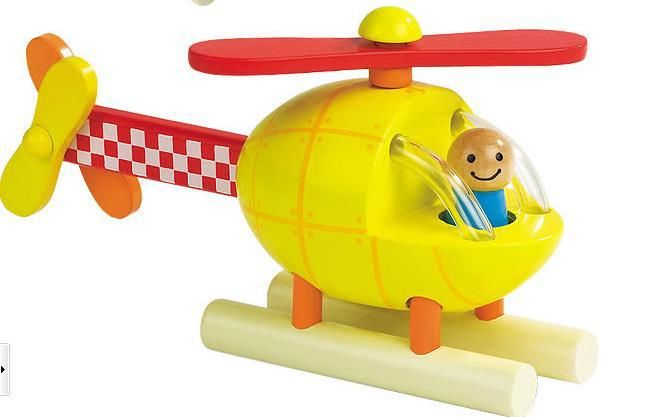In the image, a vibrant children's toy helicopter is featured prominently against a white background. The main body of the helicopter is primarily yellow, adorned with orange panel lines and orange dots marking the corners of square panels. The top features a bold red propeller secured by a rounded yellow button-like piece. Extending from the rear of the helicopter is a checkered tail with alternating red and white squares, leading to two additional rotors at the tail's end, one yellow and one orange.

The helicopter is designed to include a smiling pilot figure, whose round wooden head features black eyes and a cheerful expression. This figure, donning a blue shirt, is seated within the helicopter's main compartment, protected by two clear curved bars emerging from cutouts in the yellow body.

Supporting the helicopter are two cream-colored floats, each connected by orange legs, hinting at the toy's ability to mimic water landings. The detailed and colorful design of the toy, coupled with the friendly pilot, makes it a charming and engaging plaything for children.